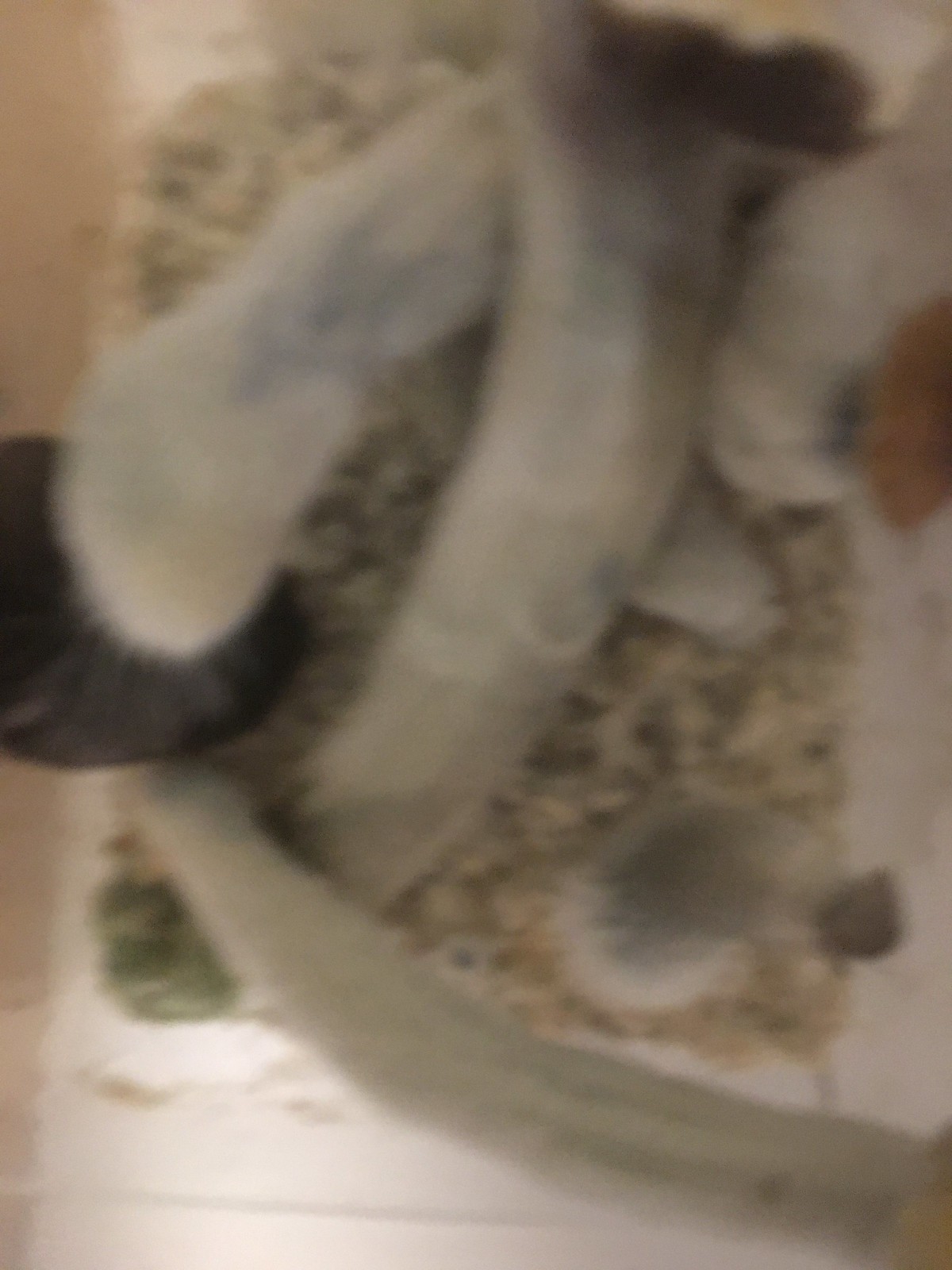In this image, captured from a top-down perspective, an assortment of white and gray objects, which somewhat resemble bones, are scattered across a white surface, possibly a tray or flat table. These objects are densely packed and overlap each other, contributing to an intriguing visual complexity. Below the larger, bone-like items, there are smaller fragments that appear to be either white or tan, though the image’s blurriness makes it difficult to discern precise details. The scene is shrouded in an overall lack of focus, obscuring finer elements and leaving the objects' exact nature ambiguous. The surrounding area hints at being part of a larger table or workspace, yet this remains indistinct due to the pervasive blur.